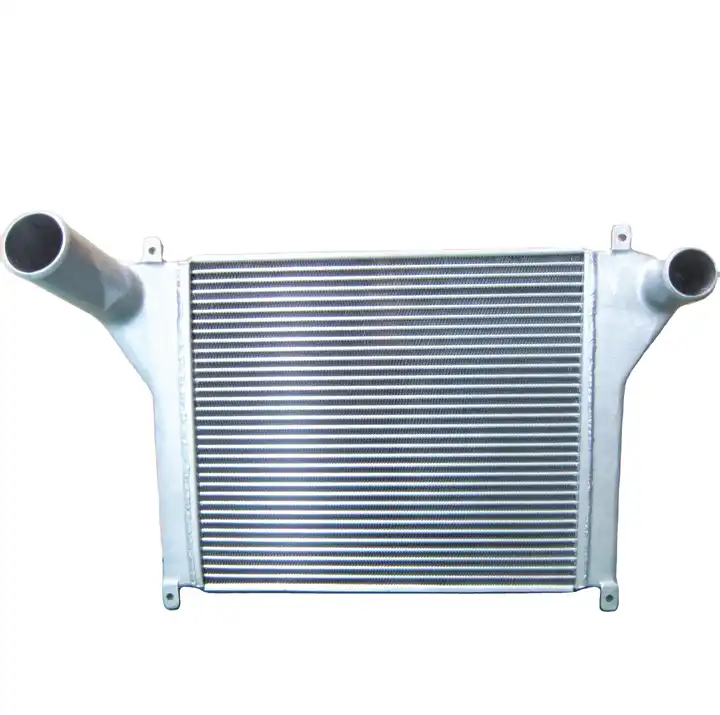The image features a robust steel piece of equipment, likely an industrial component, characterized by a central metal grate reminiscent of an air conditioner vent, with horizontal bars across its black void. The equipment is primarily painted a light gray, indicating a treatment for durability. It boasts two prominent pipe-like protrusions on both the left and right sides—used perhaps for fluid or air flow, as often seen in radiators. Additionally, the structure is designed for secure mounting with flanges at the top left, top right, bottom left, and bottom right corners, allowing it to be affixed onto walls or other surfaces. The left pipe appears longer than the right, adding to its unique design. This heavy-duty part, presented against a stark white background, suggests it's intended for detailed, technical applications such as in industrial parts stores or wholesale inventory systems, hinting at its critical role in machinery or HVAC systems.